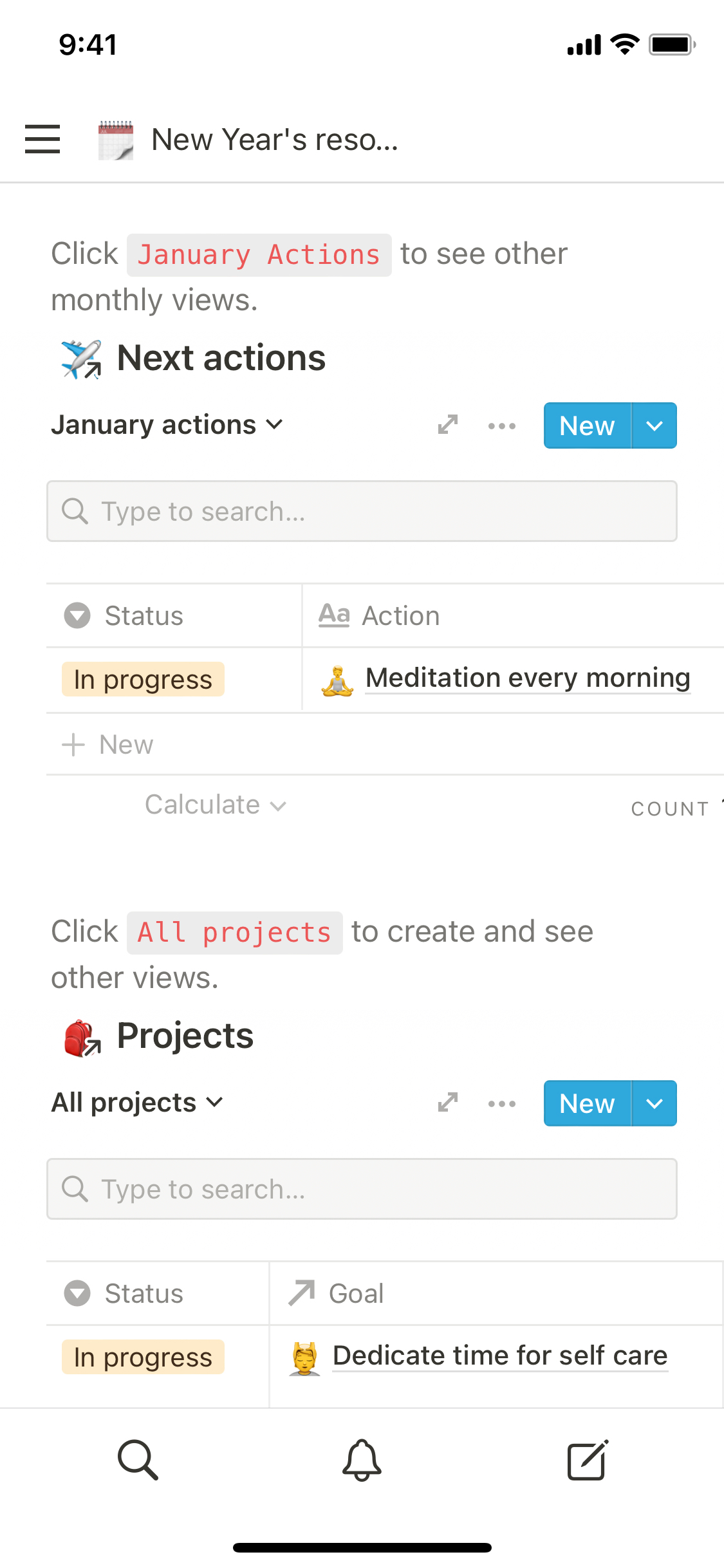Vertical smartphone screenshot depicting a productivity app interface. The screen is positioned against a plain white background, likely the computer screen's backdrop. 

- **Top Section**:
    - **Time**: Bold black text displaying '9:41' at the top left.
    - **Status Indicators**: Icons for full cellular bars, Wi-Fi signal, and battery life at the top right.

- **Main Content**:
    - **Header**: Underneath the time, three horizontal lines followed by a calendar entry:
        - **Calendar Entry**: "New Year's Reso..." separated by gray lines. This likely indicates a New Year's Resolution.
    - **Actions Section**:
        - Text instructing users to "Click January Actions" and in a red rectangular box, it reads "see other monthly views."
        - An airplane icon signaling the "Next Sections" in black text.
        - **Action Header**: "January Actions" in bold black text.
        - Option to "Click on New" and "Type to Search."
        - **Status**: Highlighted status indicating "In Progress."
        - **Action Item**: "Mediation (or Meditation) Every Morning."

- **Additional Features**:
    - Buttons labeled "Plus New," "Calculate," and "Count."
    - Another clickable gray box with the red text "All Projects" to create and view other projects.

- **Projects Section**:
    - **Icon**: A small icon next to the bold black text "Projects."
    - **Dropdown**: "All Projects" with an arrow symbol indicating a dropdown menu.
    - Options to "Click on New" and "Type to Search."
    - A gray icon labeled "Status" specifies the status as "In Progress."
    - **Goal**: "Dedicate Time for Self-Care."

- **Bottom Section**:
    - Three icons including a search engine icon, a bell, and a writing pen inside a square, with a black line running at the bottom of the screen.

This detailed caption thoroughly describes the interface elements and functionality visible in the screenshot.